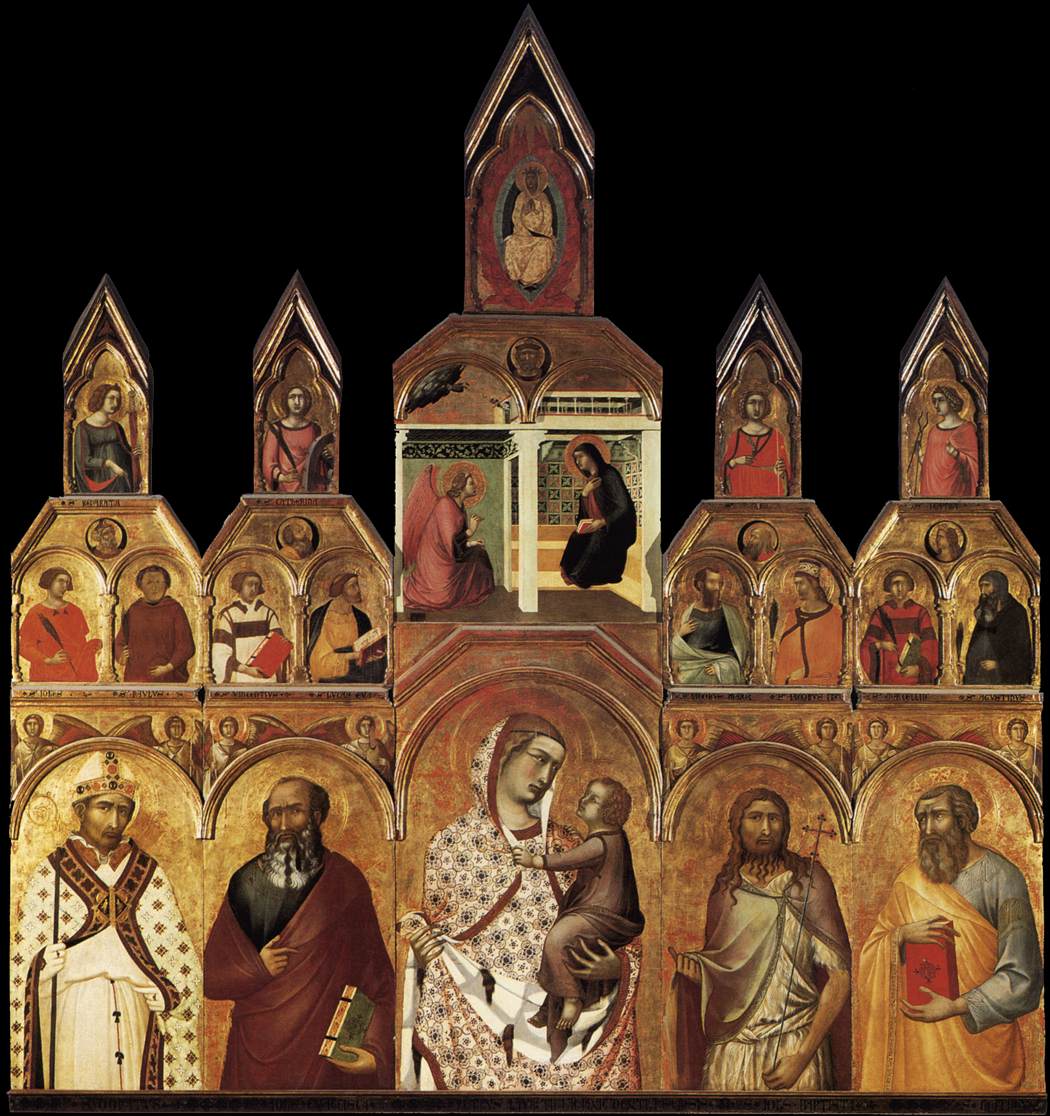This large square image showcases a Renaissance polyptych by Italian artist Pietro Lorenzetti, painted in tempera and gold. The scene is a facade reminiscent of a medieval church, cut open to reveal its interior filled with figures dressed in ancient, Renaissance-style outfits. The background is predominantly black, accentuating the ornate and intricate structure that dominates the composition.

At the bottom center, the Madonna, a woman draped in white with red and blue embroidery, holds a child clothed in brown. She is flanked by men dressed in various robes - white, burgundy, and gold. Notably, the man in the lower right corner holds a red book. Above this central group, the building rises, adorned with arches, each containing figures in different poses and attires. There are four figures on each side of the middle section and two at the tower's peak, making a total of 18 individuals. The structure features five distinctive rooftops, with the central peak being the tallest, soaring high with a sharp, angular point.

The color palette includes rich gold, brown, red, and hints of white and yellow, adding to the grandeur and depth of the scene. The overall effect is a detailed and vibrant depiction of biblical figures and saints, housed within an architecturally complex and beautified setting.